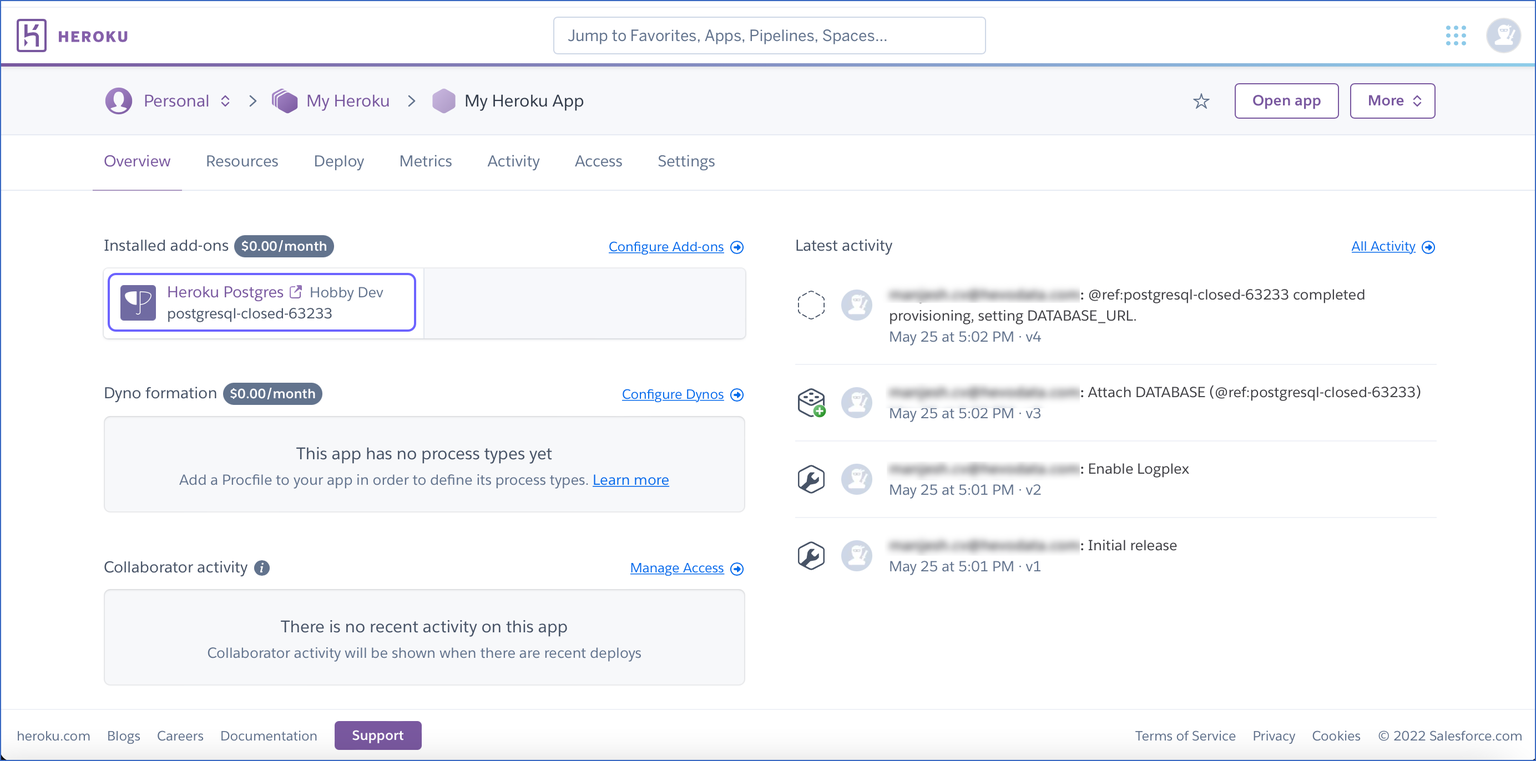Screenshot of Heroku Web Page:

The screenshot captures the Heroku web page, characterized by an overall white background. In the top-left corner, there's a prominent white square with a purple border, encompassing a large purple "K." Immediately to the right, in bold purple capital letters, it reads "HEROKU."

At the center of the page, a gray search bar displays the text “Jump to favorites, apps, pipelines, spaces...”. On the left side of this bar, a gray circle contains a white, generic person icon where a photo would typically be.

Situated below, a 3x3 grid of blue dots forms a square pattern. Encompassing this section is a thin purple border, followed shortly by a faint blue border just beneath the “KU” in “HEROKU.”

Below this, there’s a purple circle with another person icon inside, labeled "Personnel." Next to it, a diamond-shaped icon labeled "MyHeroku" also appears, accompanied by smaller fading diamonds and the text "MyHeroku App."

On the right side, a white tab with a purple border reads "More," followed by another tab that says "Open App."

Shifting focus to the left side, directly under "Personnel," a white-bordered section features the words "Overview" in purple, then "Resources" in black, followed by "Deploy," "Metrics," "Activity," "Access," and "Settings."

Below, a section titled “Installed Add-ons” includes information on additional services. On the right, a blue option labeled "Configure Add-ons" is visible. Further down, there's "Dyno Information" with a corresponding "Configure Dynos" blue option. The "Collaborator Activity" section states "Manage Access," and adjacent to it on the left, "Latest Activity" is noted, while on the right, in blue, it says "All Activity." Beneath, there are four profile icons and accompanying text.

At the bottom left corner, the purple text reads "Heroku.com" followed by “Blogs” and “Careers,” then "Documentation." A purple tab here states "Support" in white.

Finally, on the bottom right side, it mentions “2022 Salesforce.com” followed by links for “Cookies,” “Privacy,” and “Terms of Policy.” 

This detailed layout encapsulates the main elements and visual structure of the Heroku web page.